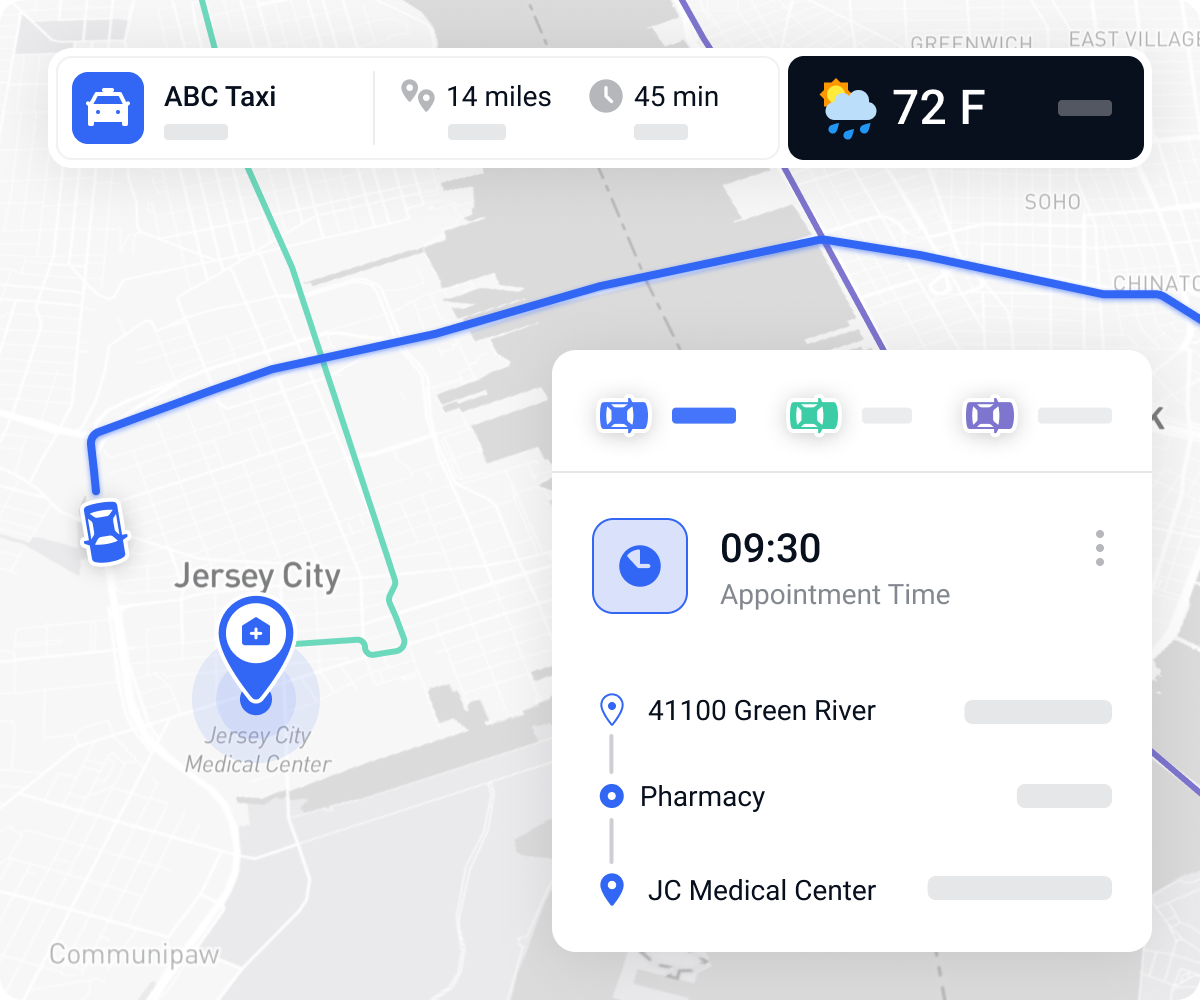The image is a detailed map displayed on a device, most likely a smartphone. At the top, a blue square with a white taxi icon is labeled "ABC Taxi," and the map indicates that the destination is 14 miles away. Next to this, "45 minutes" is noted beside a clock icon, suggesting the estimated travel time. 

In a black rectangle at the top of the map, the weather is displayed with "72°F" alongside an icon of the sun partially obscured by a cloud with rain, indicating mild and rainy conditions.  

A car icon, depicted in blue, is positioned on the left side of the map, illustrating the route: it moves upwards, turns right, and extends across the map, exiting on the right. A pin marker in Jersey City identifies the "Jersey City Medical Center." There is a green line emanating from this area, directing northward, likely representing a route or boundary. 

In the middle section of the map, a rectangle outlines critical information, showing a "9:30 appointment time." It details the starting point at "41100 Green River," connects to "JC Medical Center," and concludes at the "Pharmacy."